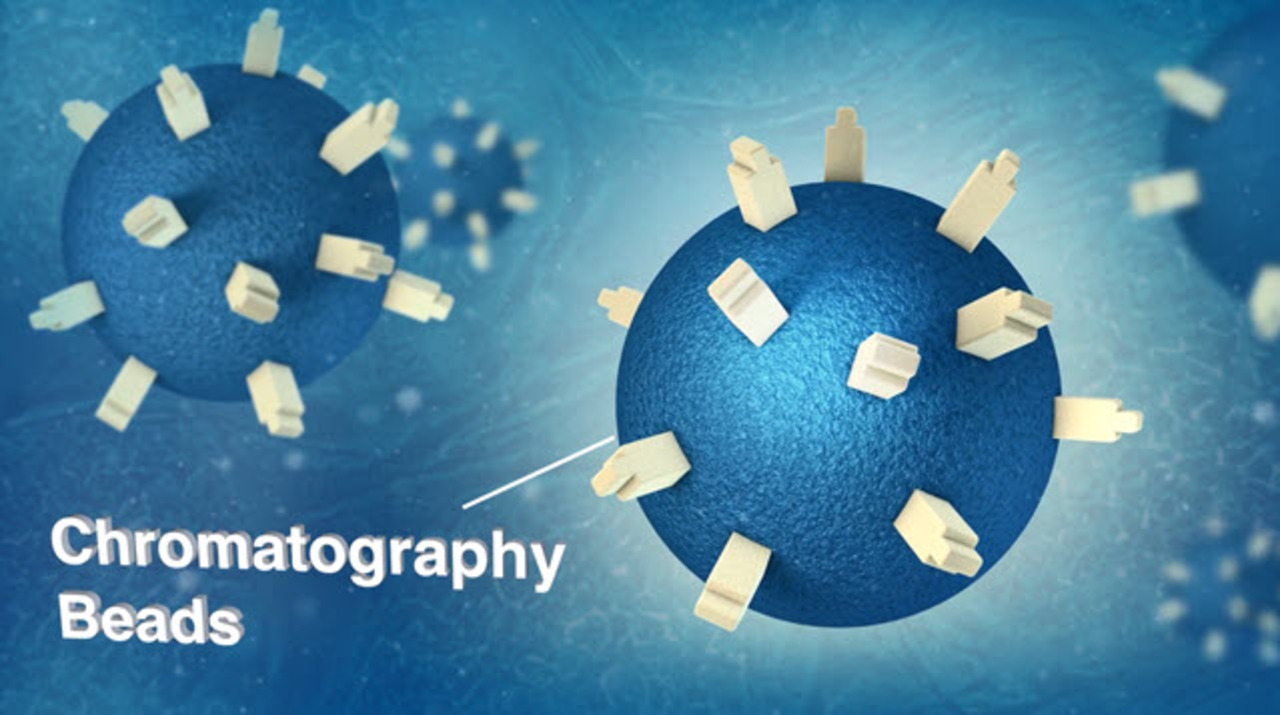This computer-generated image, formatted in a horizontally aligned rectangle, features a blue and white blended background with the phrase "chromatography beads" written in large white letters in the lower left-hand corner. The central focus is on two blue, textured, spherical objects adorned with evenly dispersed white, vertical, rectangular spikes with smaller rectangular tips at their ends. One sphere is prominently positioned on the middle right side, presented in sharp detail, while a slightly smaller sphere is situated in the upper left-hand corner, appearing less focused but similar in structure. Additionally, the background includes at least three more of these spherical objects, all blurred to convey depth, with one partially visible in the upper right-hand corner. A white line points to the central, more defined sphere, emphasizing its importance in the composition.